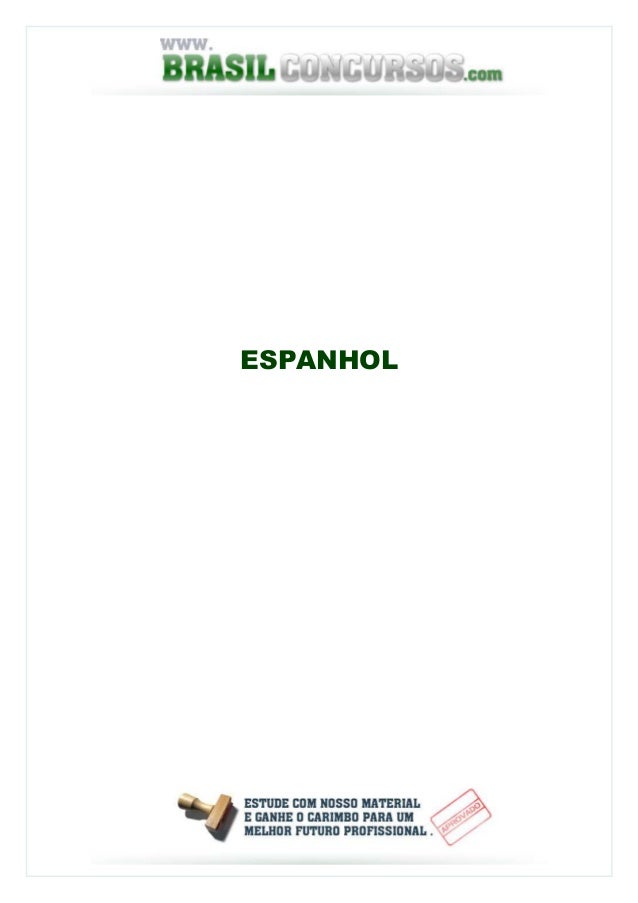The image depicts a clean, primarily white background featuring various detailed text elements. At the top, there is a web address, "www.brazilconcursos.com," with "www" in grey lowercase font, "brazil" in prominent green font, "concursos" again in a gradient grey that transitions from white at the top to grey at the bottom, and "dot com" in green. Centrally, the word "Español" appears in bold green font. The image's lower section showcases blue text stating "Estude com nosso material e ganhe o carimbo para um melhor futuro profissional." Flanking this text, on the left, is an illustration of a brown stamp tilted on its side, and on the right is a silver representation of a stamp marked "Aprovado." The overall impression is that of a potentially educational or professional manual, emphasizing approval and quality material for Spanish-speaking users.